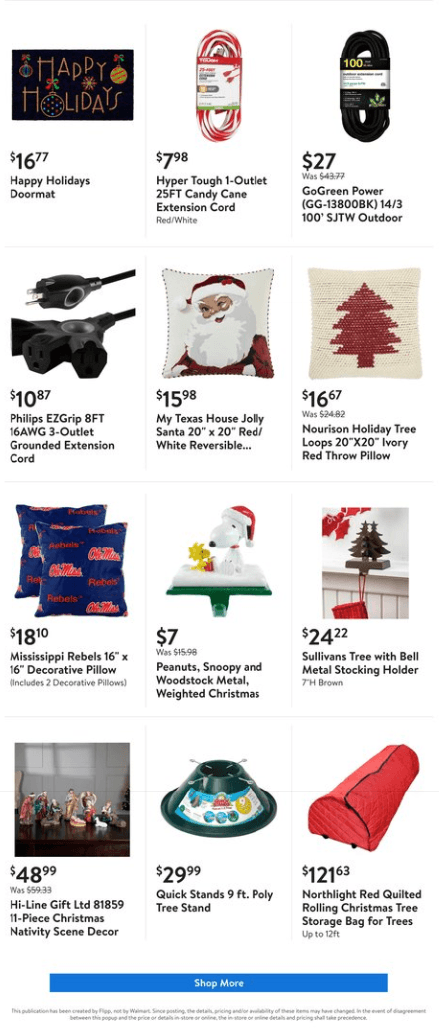This image is a screenshot from a smartphone displaying an online store interface with various holiday-themed items for sale, organized in a grid of rows and columns. 

At the top, prominently featured is a "Happy Holidays" doormat priced at $16.77. To its right is a Hyper Tough One Outlet Candy Cane Extension Cord, listed for $7.98. Adjacent to that, another listing titled "Go Green Power Outdoor" displays a black extension cord priced at $27.

In the subsequent row, starting from the left, there is a Phillips Easy Grip 8-Foot Grounded Extension Cord selling for $10.87. Centered in this row is a My Texas House Jolly Santa 20x20 Red and White Reversible Pillow, retailing at $15.98. To the right, a Norrison Holiday Tree Loops Ivory Red Throw Pillow is displayed at $16.67.

Further down, there are two additional rows, each containing three boxed items with their respective prices clearly visible. 

At the very bottom of the screen, a blue rectangle button invites customers to "Shop More."